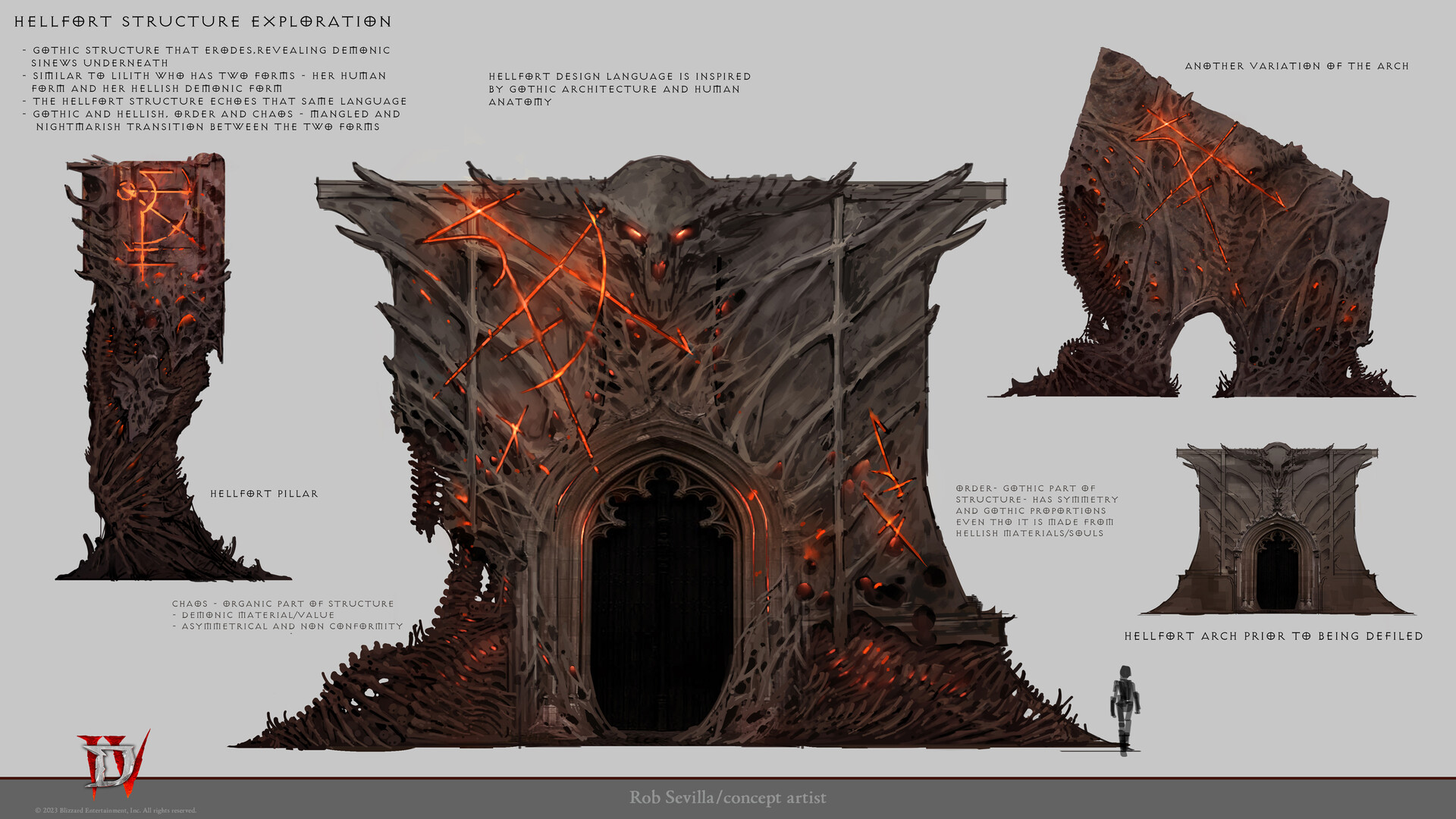This concept art depicts a large, demonic-looking fantasy building known as the Hellfort, a structure that embodies a nightmarish fusion of gothic and hellish designs. At the center of the illustration stands a towering flat building with a giant horned skull featuring glowing orange eyes at the top. The skeletal sides of the edifice are etched with menacing, orange rune flames, and the imposing structure includes a large, gaping black doorway at its base. The layout includes detailed side and back views, along with numerous elements annotated with descriptive text. 

In the top left corner, the label "Hellfort Structure Exploration" suggests a deep dive into the architectural and thematic elements of the building. Annotations describe the Hellfort as a gothic structure revealing demonic sinews underneath, similar to the dual forms of Lilith—both her human and demonic aspects. This duality is mirrored in the Hellfort's design, blending order and chaos through its gothic and chaotic, organic parts. A pillar inscribed with fiery lines, labeled "Hellfort Pillar," is highlighted as part of its chaotic, asymmetrically designed foundation, made from demonic materials and souls.

Adjacent notes describe an "Order Gothic" part of the structure, emphasizing its symmetry and gothic proportions despite being composed of hellish substances. The depiction includes a "Hellport Design Language," inspired by gothic architecture and human anatomy. Other variations of the structure feature gates and arches, one showcasing a pristine form labeled "Hellfort Arch prior to being defiled." Additionally, the base of the building is supported by bone-like shapes and spikes that appear to be crafted from bones. The concept artist for this intricate illustration is credited as Rob Savilla.